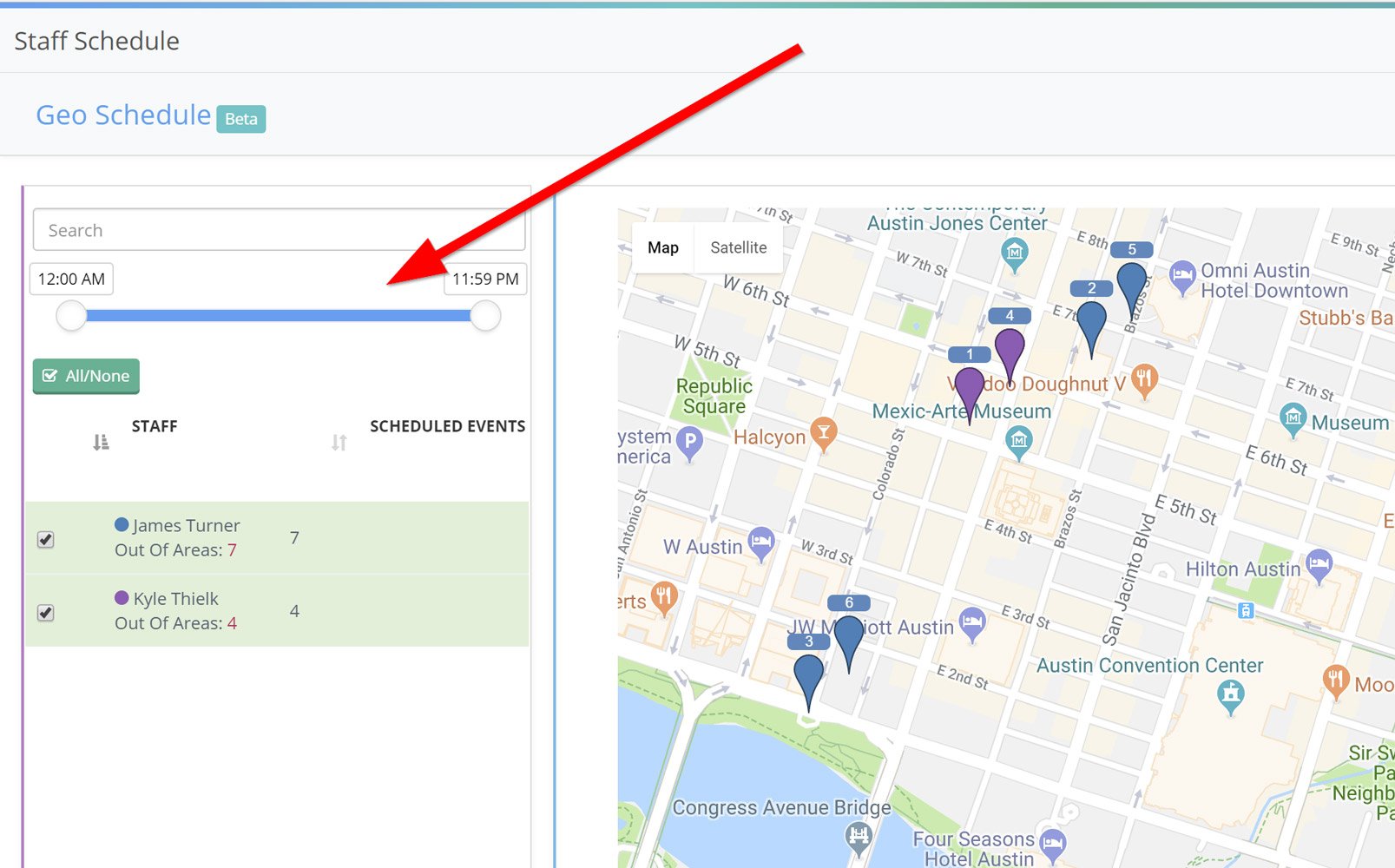The image displays a detailed layout of a scheduling interface.

At the top left, the words "Staff Schedule" are prominently displayed in black. Directly below, in blue text, it says "Geo Schedule," accompanied by a green shaded box with "Beta" written in white inside it. Below this, there is a search bar labeled "Search."

The time range is indicated with "12 a.m." on the left and "11:59 p.m." on the right, suggesting that these times can be adjusted. A blue horizontal line stretches across, ending in small white circles on both ends. A prominent red arrow points towards the right end of this blue line.

Beneath the blue line, on the left, there is a white check box with the text "All or None" in a green banner. Below this, the sections "Staff" and "Scheduled Events" are marked against a white background.

Towards the bottom, a gray-shaded background lists individual staff members and their availability. "James Turner" is mentioned as being out of area 7, indicated by a green circle with the number 7 in purple. "Kyle Field" is out of area 4, marked by a purple circle, with the number 4 in purple.

To the right of these details is a Google Map interface showing icons and location markers in blue and purple. Key locations and events on the map include "Voodoo Donut," "Mexic-Arte Museum," "Omni Austin Hotel Downtown," "Marriott Austin," "Halcyon," and "System America," each marked with respective icons.

This detailed interface appears to combine staff scheduling with geographic location tracking, providing a comprehensive tool for managing events and personnel.